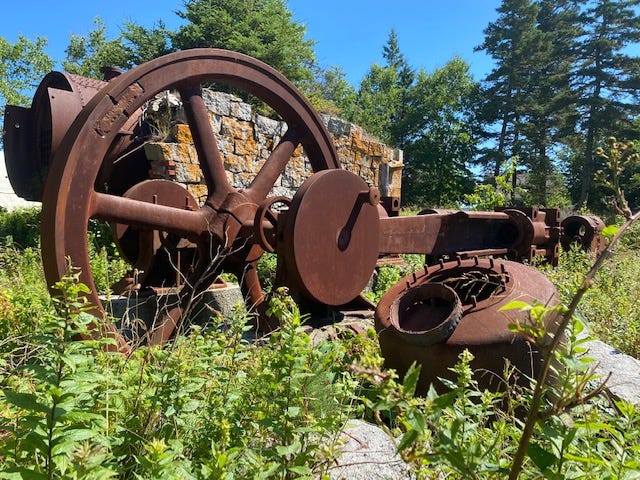The photograph captures an outdoor scene featuring an old, rusted cannon or piece of machinery resting amidst high green brush and tall weeds. The dark brown, weather-worn metal structure has a central wheel with a turnable handle, and several of its components are scattered around. In the foreground, among the green and slightly yellow grass, a prominent rock is visible. A rock walkway extends off from the right, leading up to the cannon, which is oriented to the right side of the image. Behind the cannon, there is a rustic brick wall composed of gray and rust-colored bricks. The background is filled with tall, green-leaved trees that surround the area, and the clear blue sky with no clouds above, illuminated by the shining sun, completes this picturesque scene.